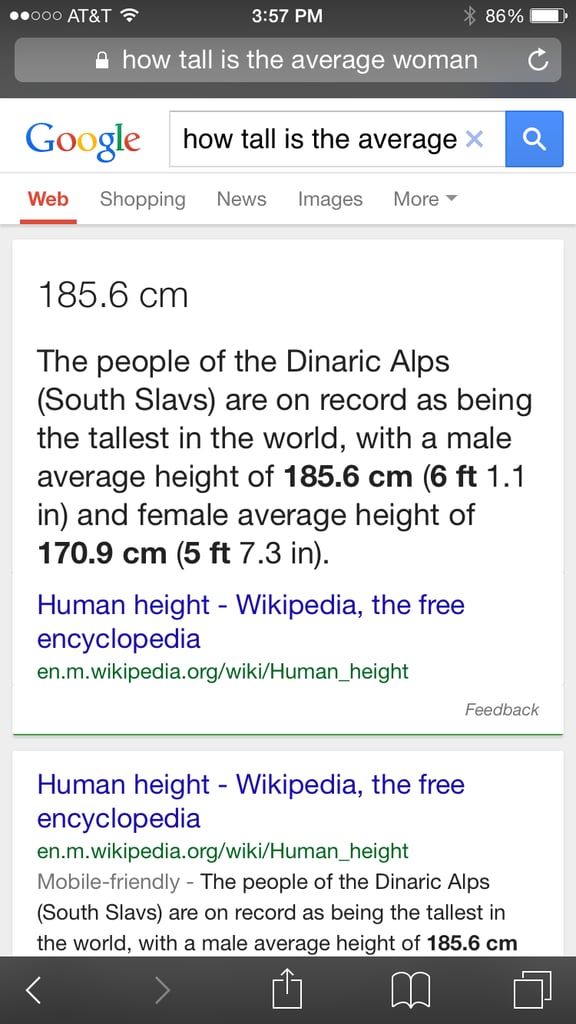This image is a screenshot of a cell phone displaying a Google search result page. The phone's interface features a white background framed by black bars at the top and bottom of the screen. Within the top black bar, on the left, two out of five round dots indicate the cellular connectivity strength, followed by a label "AT&T" and a Wi-Fi signal icon. Centered in this bar is the current time, 3:57 p.m., while the right side shows an 86% battery level alongside a nearly full battery icon.

In a gray search bar toward the top of the screen, featuring a white lock icon on the left and a refresh button on the right, the query is, "How tall is the average woman?" Directly below this is the colorful Google logo, accompanied by the search query repeated in a smaller search bar containing an 'X' icon and a blue magnifying glass icon to initiate the search.

Immediately below this bar are five selectable tabs: Web (highlighted in red and underlined), Shopping, News, Images, and More. The Web tab is currently selected. 

The first result appears in a gray highlight box and begins with a numerical value: "185.6 centimeters." The description below this states: "The people of the Donarik Alps South Slobs are on record as being the tallest in the world, with a male average height of 185.6 centimeters (6 feet, 1.1 inches) and a female average height of 170.9 centimeters (5 feet, 7.3 inches)." This result is attributed to "Human height - Wikipedia, the free encyclopedia," with the web address shown below in green text.

The second entry, labeled "Human height - Wikipedia, the free encyclopedia," has a blue hyperlink to the article and repeats the information from the first result. The web address is shown beneath it and is marked as "mobile-friendly."

The bottom black bar of the screen features five icons: a left arrow to go back, a right arrow to advance, a download box, a bookmark icon, and an icon for multiple screens. This screenshot comprehensively showcases a Google search on the average height of women, highlighted by details of the cell phone interface and search results.